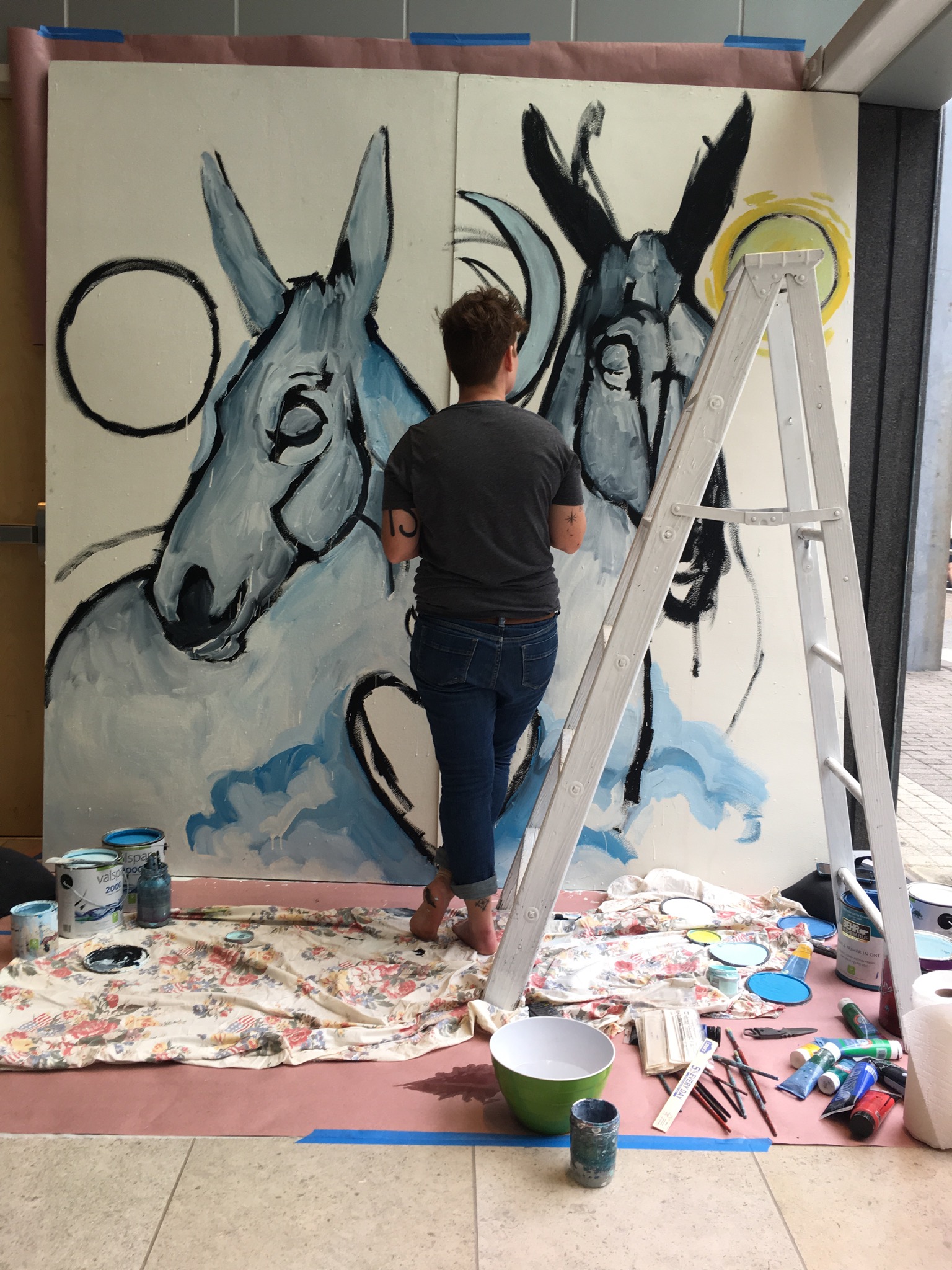This photograph captures a scene of an artist deeply engrossed in her work on an impressively large canvas, which stands taller than she does. The artist, barefoot, dressed in blue jeans and a grey short-sleeve t-shirt that reveals hints of tattoos on her upper arms, is viewed from behind. With short brown hair cascading just above the nape, she stands with her legs crossed in a moment of contemplative focus before her canvas.

The canvas itself, stark white and possibly divided into two halves, dominates the art studio. The artwork features two horse heads rendered in early stages of blue, grey, and black hues. Each horse head faces opposite directions, with one pointing left and the other right. The upper right corner of one side of the canvas contains a depiction of a sun, while the upper left corner of the other side features a circle that might also be a sun in progress.

Surrounding the artist is an organized chaos typical of a creative space—pink paper is laid out on the floor to protect it, accompanied by a silver ladder positioned to the artist's right. To the left, cans of paint are placed, with numerous paint brushes, tubes of paint, and lids scattered on the floor under the ladder. This immersive environment frames the artist's labor and dedication as she works to bring her vision to life.